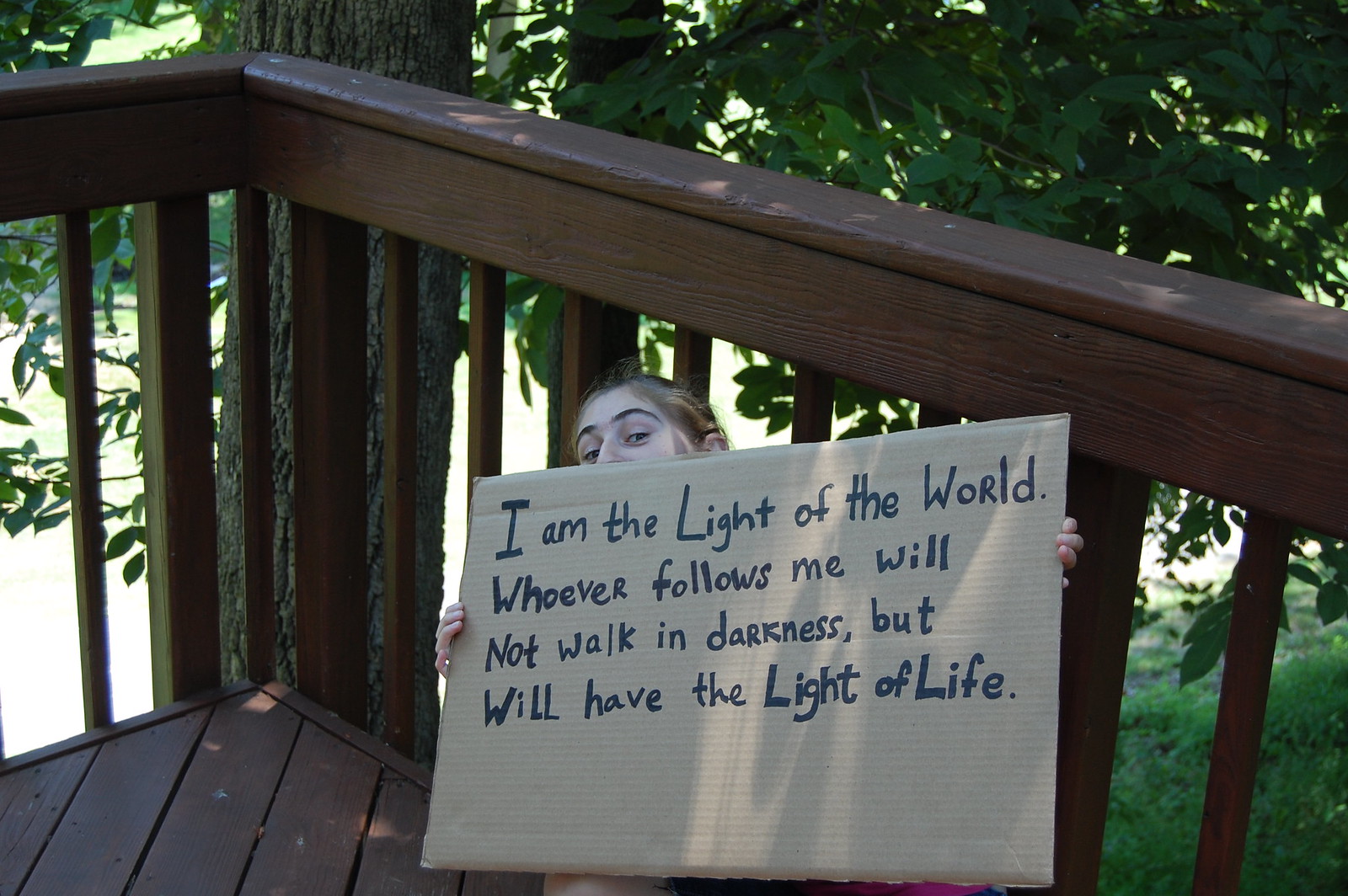In this outdoor photograph taken on a porch or balcony, a young girl with chestnut brown hair pulled back and dark eyes peeks over the top of a cardboard sign she is holding. The sign, printed with a black marker, reads: "I am the light of the world. Whoever follows me will not walk in darkness but will have the light of life." The porch is made of wood with a dark stain, and behind it, a large tree with lush green leaves can be seen. The ground below is covered with grass and other vegetation. The girl, who appears to be crouching or sitting down, holds the sign with both of her small hands, making for a scene that highlights the colors brown and green. The image, likely taken by a family member, has a serene and slightly religious tone.